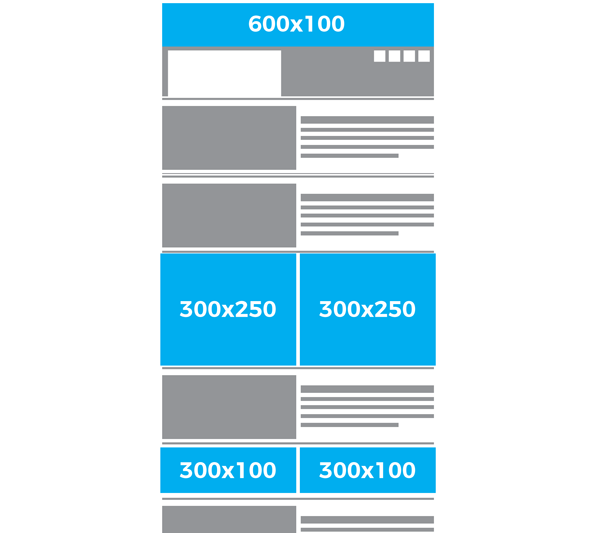This vertical rectangular image is meticulously organized with various sections and labels. At the very top is a blue banner stretching across the width, with white text displaying "600 x 100." Below this banner are three separate boxes adorned with a mix of gray and white shapes, each box demarcated by horizontal lines, collectively filling up the top half of the image.

Midway down, the layout changes to feature two prominent blue boxes that span the entire width side-by-side. The left box contains white text reading "300 x 250," while the adjacent right box displays "300 x 250." A slim vertical white line distinguishes these two sections. Immediately beneath these, a gray border acts as a divider.

Continuing downward, the next section incorporates another area with a pattern of gray and white lines, followed by another slim border. Finally, at the bottom of the image, an additional set of two blue boxes appear side-by-side, each carrying the label "300 x 100" in white text. These two boxes are also separated by a thin white vertical line. The layout concludes with a thin gray line underlining this final section, creating a structured, segmented appearance throughout the image.